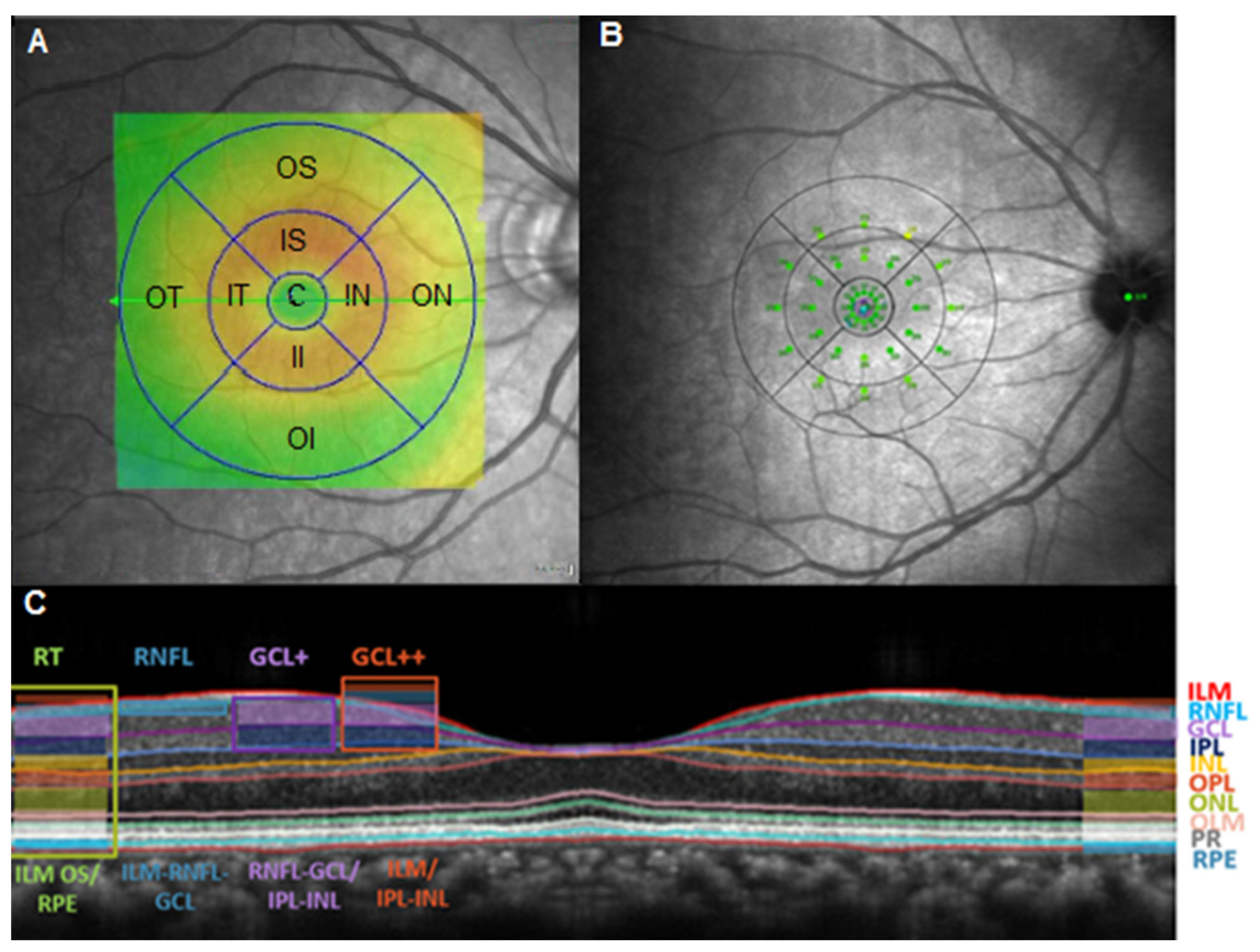This image comprises three different scientific diagrams labeled A, B, and C, all set against a black background with varying line patterns reminiscent of veins or an eyeball structure. 

In Image A, we see a detailed background of black, white, and gray lines resembling an eye, overlaid by a green and yellow box containing a circle graph. This circle is divided into eight quadrants labeled with two-letter phrases: OS, ON, OI, OT occupy the larger quadrants, while IS, IN, II, IT fill the smaller ones. In the center of the circle is a smaller circle marked with "C."

Image B displays a similar vein-like background but features a transparent circle with green dots inside it, continuing the theme of anatomical detail.

Lastly, Image C depicts a color spectrum graph with overlapping, mountain-like waves representing different data codes, including RT, RN, FL, GCL+, GCL++. This part of the image emphasizes the variations in the color-coded data, arranged in a wavelength pattern.

Together, these diagrams analyze complex scientific data, possibly related to an eye scan or similar medical imaging technology.